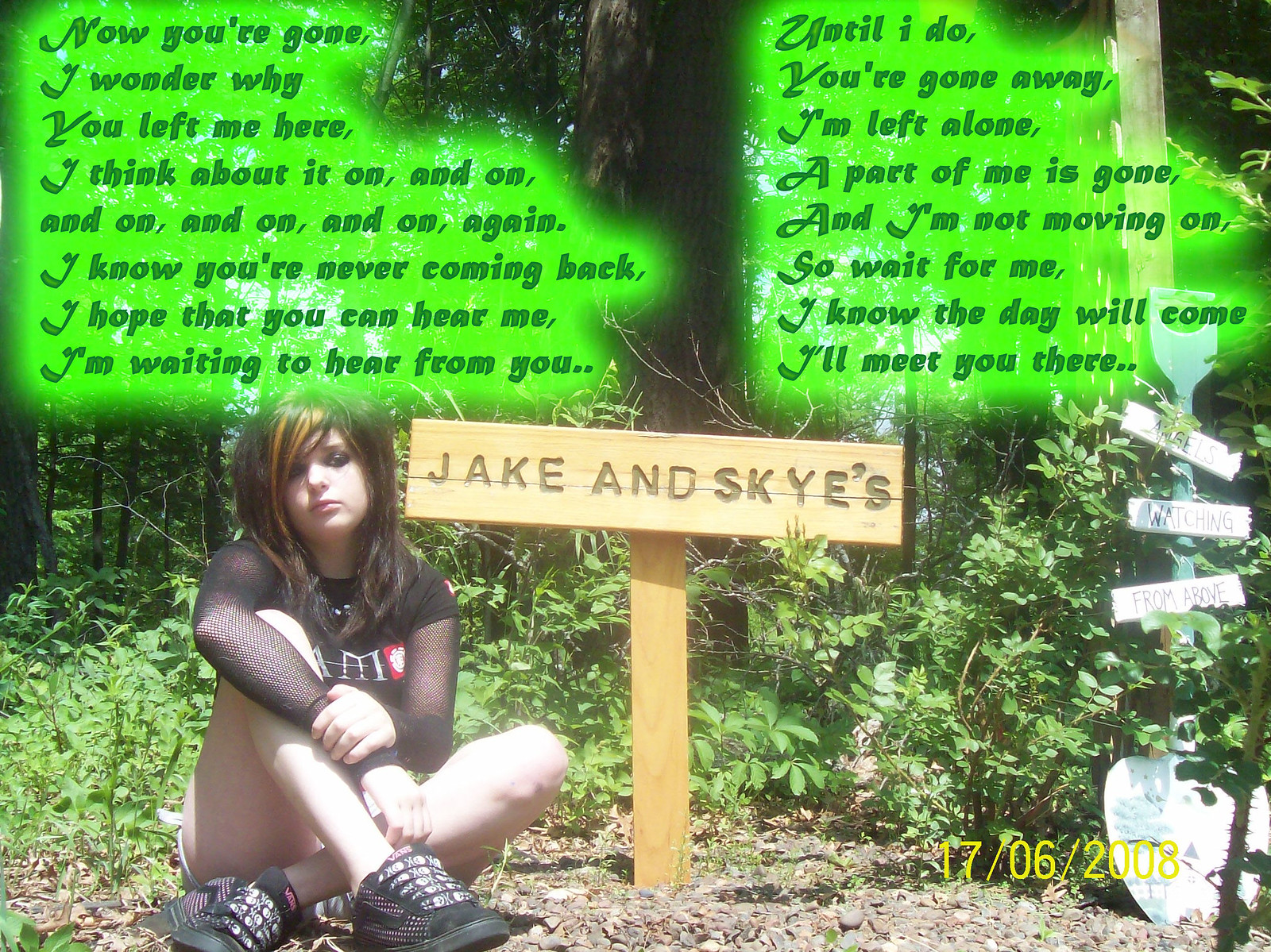The image depicts a young, emo-looking girl with black hair, dressed in a black lace mesh shirt, black shorts, and black tennis shoes. She is sitting on the ground, which appears to be dirt, next to what looks like a makeshift grave marked by a wooden cross made of two-by-fours, with the name "Jake" inscribed on it. In the bottom right corner, the date "17-06-2006" is visible. The somber setting is accentuated by a neon green overlay at the top, featuring an emotional poem. The poem reads: "Now you're gone, I wonder why you left me here. I think about it on and on and on and on and on again. I know you're never coming back. I hope that you can hear me. I'm waiting to hear from you. Until I do, you're gone away. I'm left alone, a part of me is gone and I'm not moving on. So wait for me, I know that day will come. I'll meet you there." The image conveys a poignant tribute to someone named Jake, who has passed away, capturing the deep sorrow and longing of the girl mourning him.